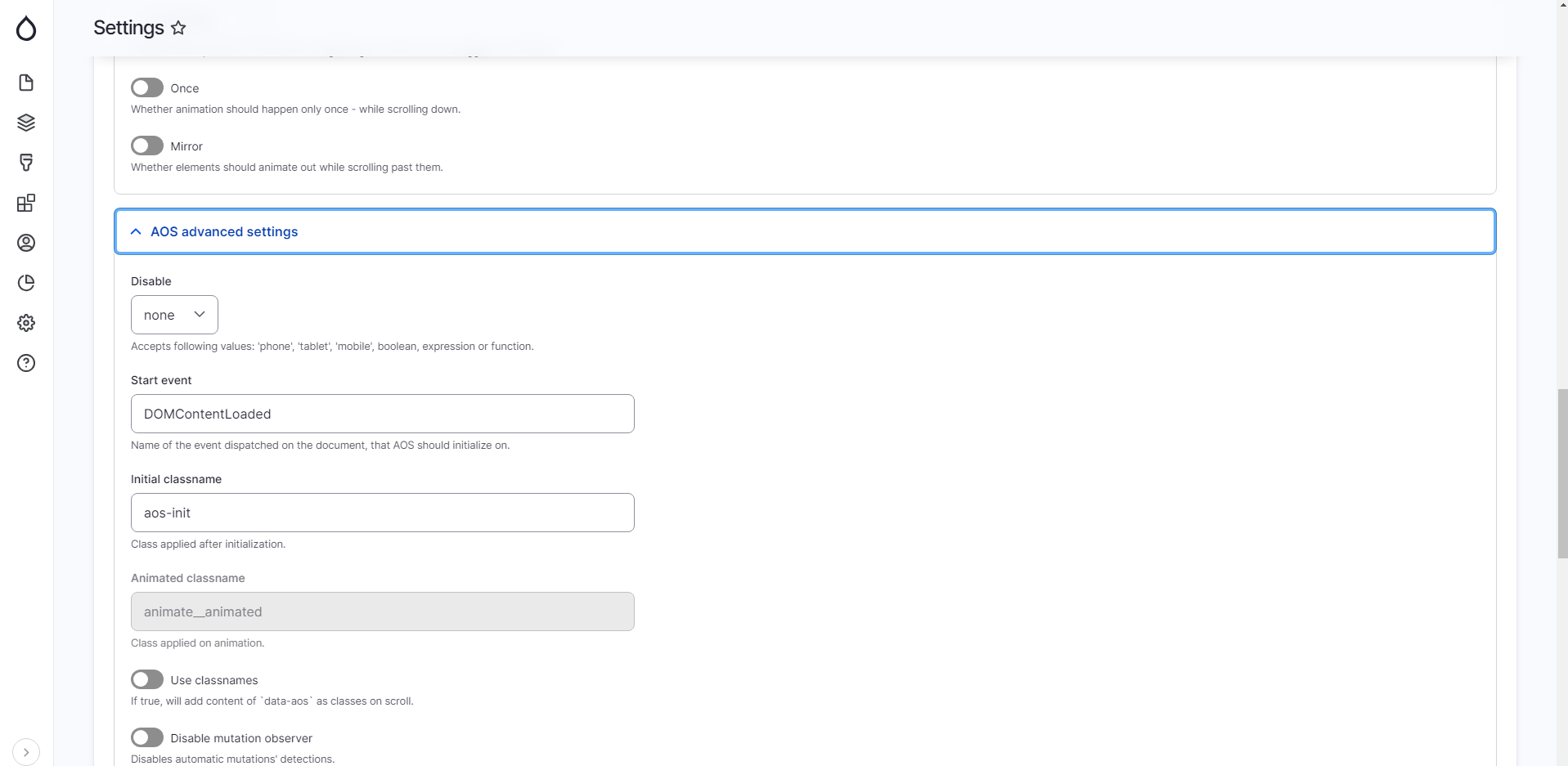A detailed screenshot of the AOS (Animate On Scroll) settings menu is displayed, surrounded by a gray frame with the title "Settings" prominently featured in the frame. 

Within the settings, two options – "Once" and "Mirror" – are listed, both toggled off. These settings determine whether animations should occur only once during scrolling and whether elements should animate as they scroll past, respectively.

Below these settings is a blue box labeled "AOS Advanced Settings." Within this section:
- **Disable:** currently set to "none".
- **Start Event:** specified as "DOMContentLoaded", indicating the event that triggers AOS initialization.
- **Initial Class Name:** set to "AOS-INIT", which is applied after initialization.
- **Animated Class Name:** set to "animate_underline animated", specifying the class applied during animation.

Additional settings include:
- **Use Class Names:** Currently off, this setting would add the content of the data-AOS attribute as classes during scrolling if enabled.
- **Disable Mutation Observer:** Also off, this setting would disable the automatic detection of DOM mutations.

Overall, this settings menu provides detailed configuration options for controlling the behavior of animations in a scrolling content environment.